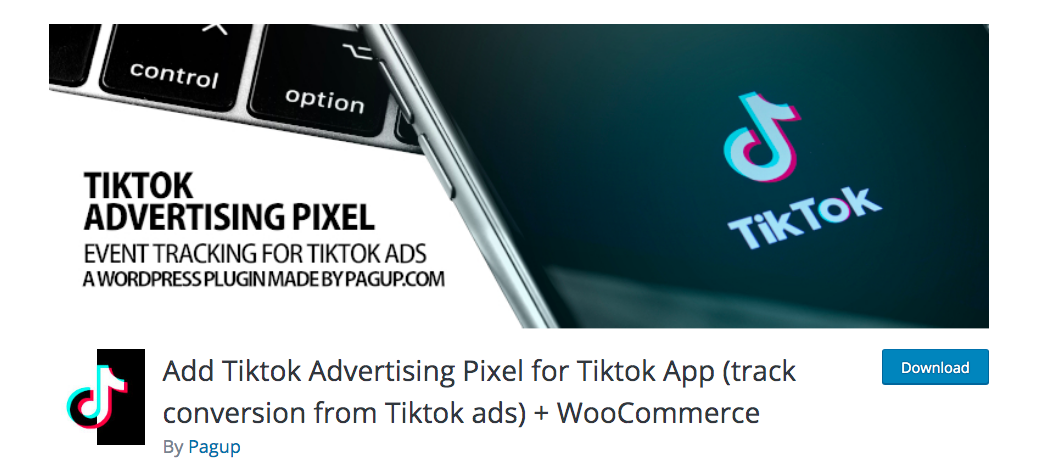This image is an advertisement for a WordPress plugin designed by PageUp.com, focused on integrating TikTok's advertising pixel with WooCommerce. Dominating the top section of the ad is the headline "TikTok Advertising Pixel: Event Tracking for TikTok Ads." Below the headline, the ad emphasizes the capability of the plugin, stating, "Add TikTok advertising pixel for the TikTok app. Track conversions from TikTok ads plus WooCommerce by PageUp."

In the center of the image, there is a partial screenshot featuring control and option buttons, overlaid with the image of a tablet displaying the TikTok logo with its distinctive pink outline on a black background, accompanied by the text "TikTok." The overall page has a white background, adding a clean and modern aesthetic to the design. At the bottom, a prominent blue download button invites users to obtain the plugin. This advertisement effectively promotes the PageUp.com plugin, which facilitates the tracking of TikTok ad events for WordPress users.